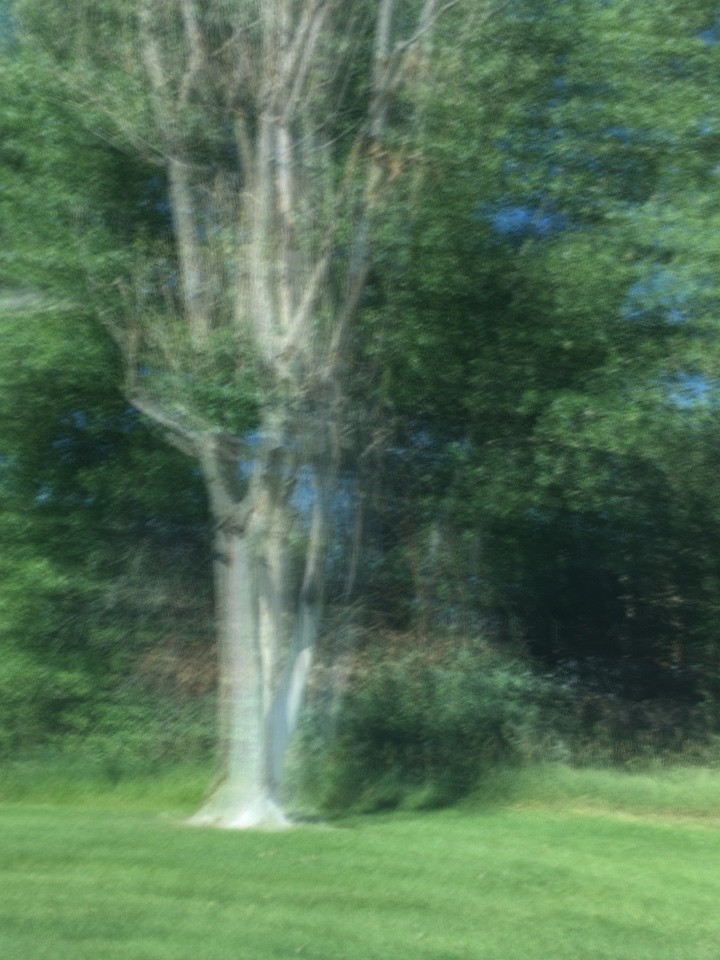In a sunlit yard or field, an intriguing image captures a leafless tree with a unique, almost holographic appearance. The tree, primarily white with hints of silver in its bark, stands on a well-trimmed grassy area. Its numerous bare branches reach upwards, with only a few green leaves sprouting near the center. The tree's blurred and duplicated effect gives it a surreal, multi-layered look. Surrounding the focal tree, dense shrubbery and additional trees form a lush green backdrop, though their trunks are obscured by the foliage. Patches of clear, vibrant blue sky peek through the leafy canopy, enhancing the impression of a bright, sunny day. Further back, taller grasses extend beyond the main scene, completing the picturesque and somewhat otherworldly landscape.